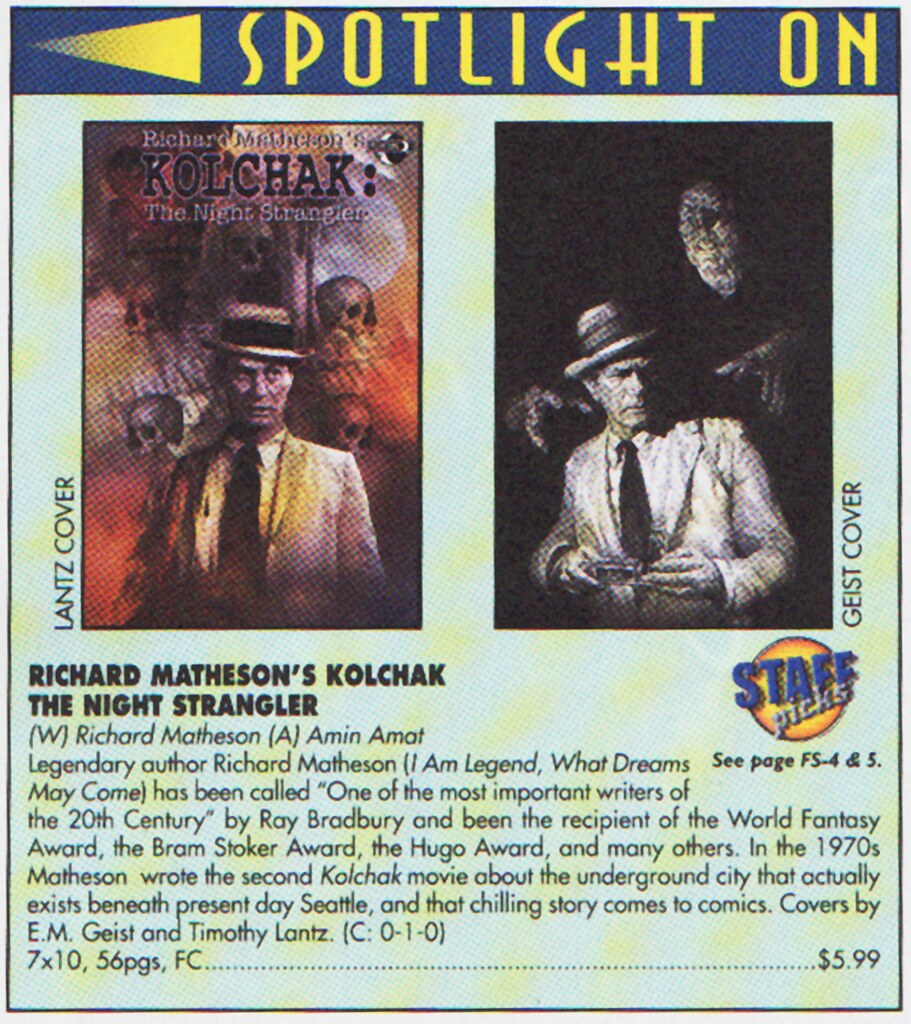The image is an old, worn poster-like advertisement that resembles a magazine or newspaper page. At the top, against a blue banner, the yellow text reads "Spotlight on," followed by an arrow pointing to the left. Below the banner are two distinct images. The left image shows a man in a white suit and top hat, standing against a red background filled with skulls, labeled "Lance cover" to the left. The right image, in black and white, features the same man, but this time a tall creature with extended hands looms behind him; this image is labeled "Geist cover."

Below these images, in bold black writing, it reads "Richard Matheson's Kolchak: The Night Strangler." There’s a descriptive paragraph mentioning legendary author Richard Matheson, known for works like "I Am Legend" and "What Dreams May Come," and noting his accolades including the World Fantasy Award, the Bram Stoker Award, and the Hugo Award. The description explains that in the 1970s, Matheson wrote the second Kolchak movie about an underground city beneath Seattle, which is now adapted into this comic book. The comic features covers by E. M. Geist and Timothy Lance, is sized 7x10 inches, and has 56 full-color pages. A dotted line at the bottom right side leads to the price, listed as $5.99. There is also an orange circle above the right image, with "staff pics" written in blue text against a yellow background.